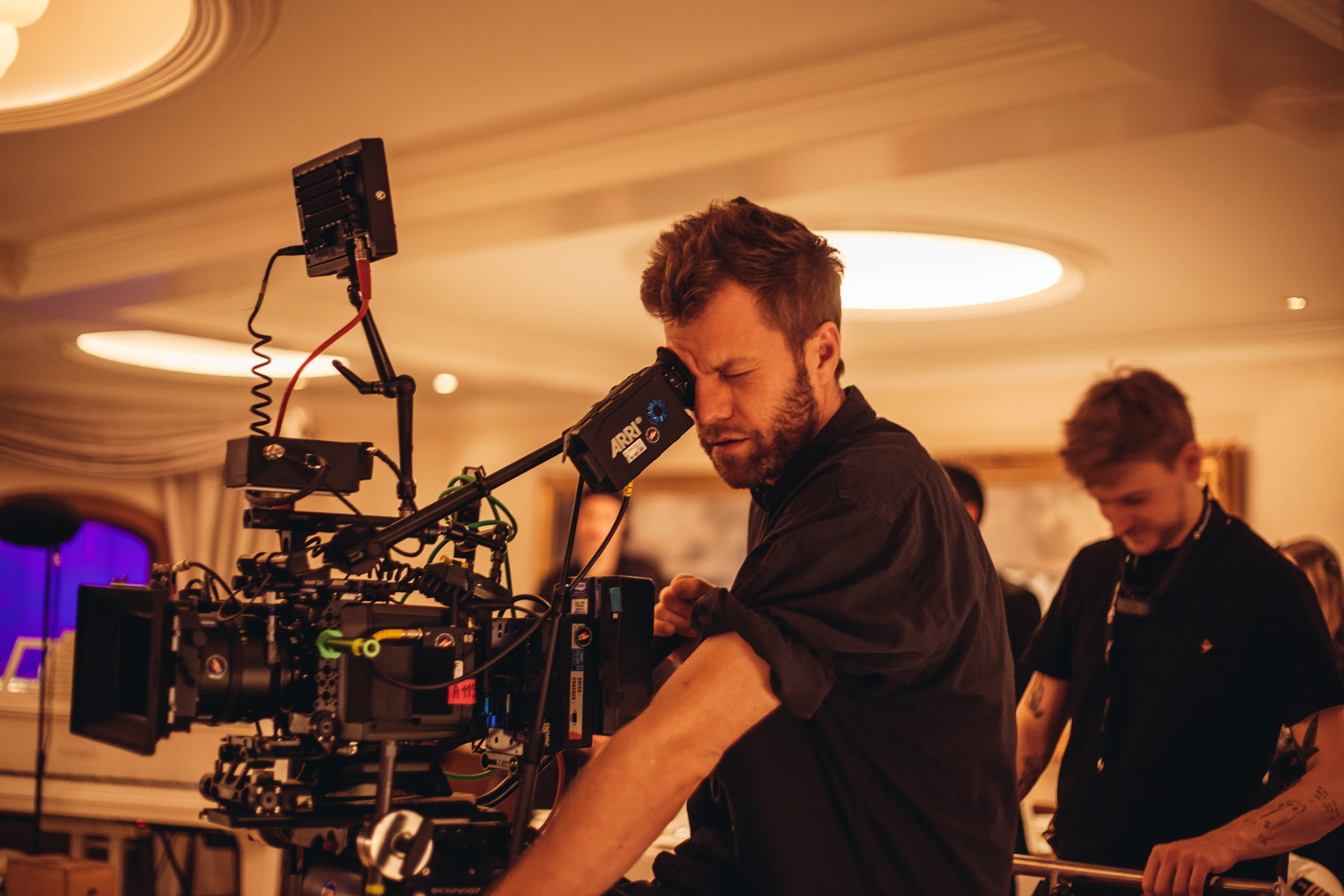This digital photograph shows a white man operating a complex, television-style camera in the center-right of the image. His face is pressed up against a separated viewfinder, his expression scrunched in concentration as he peers through the lens with one eye closed. He wears a black dress shirt with the sleeves rolled up, his right hand busy maneuvering the intricate camera, which is laden with numerous pieces and wires stretching between the main body and the lens. The camera is mounted on a tripod or stand and is aimed towards the left-hand side of the photo.

Behind the cameraman, two or three crew members, also dressed in black, are visible but their exact activities are unclear. One of these crew members is notably holding some sort of filming or recording equipment, adding to the bustling scene. The background suggests they are in a grand indoor environment, possibly a ballroom or a hotel lobby, characterized by large, round white lights on a tan-colored ceiling. The atmosphere hints at the setting of a TV show or movie production.